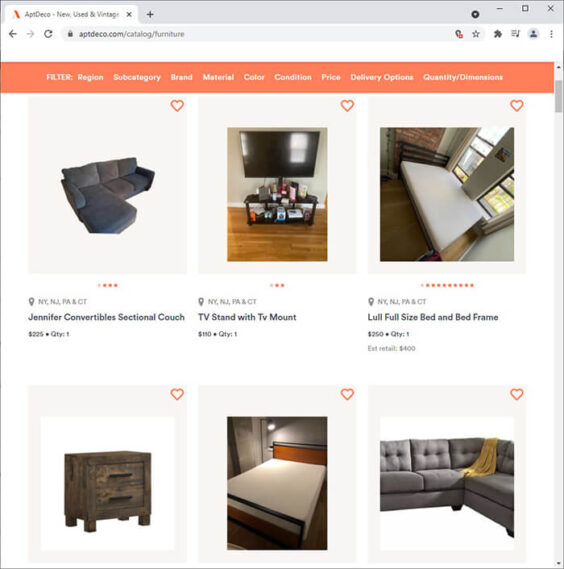This is a vertical screenshot from a computer showcasing a browsing session on a website for new, used, and vintage items. At the top, a gray navigation bar stretches across the screen, featuring a tab labeled "App Deco - New, Used, and Vintage," alongside a "+" sign to add another tab. Adjacent to this are back and forth arrows, a refresh button, a search bar, and icons, including minimize, maximize, and close (X) buttons in the upper right-hand corner.

Below the navigation bar is a white strip followed by an orange one, which includes various filter options in white text: "Filter by region, subcategory, brand, material, color, condition, price, delivery options." On the far right, a vertical scroll bar indicates the page position, currently at the top.

The main body of the page displays six product images arranged in two rows of three. Each image features a heart icon in the upper right-hand corner to favorite the item. The information beneath the top row of images provides details such as star ratings, location, item name, price, and quantity. For example, the first item is a "Jennifer Convertible Sectional Couch" with a four-star rating, located in New York, New Jersey, Pennsylvania, and Connecticut, priced at $225, and available in a single quantity. The bottom row also shows three images, but the accompanying information is cut off and not visible in the screenshot.